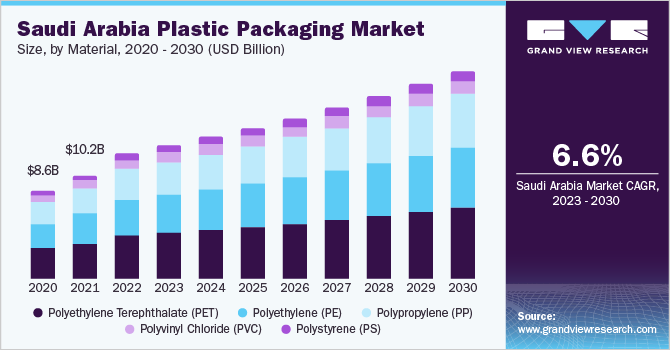The image is a detailed infographic illustrating the Saudi Arabia plastic packaging market from 2020 to 2030. The graph has an oblong horizontal shape, edged in light blue at the top against a light blue background. At the top, in bold black print, it reads, "Saudi Arabia Plastic Packaging Market." Underneath, in smaller black print, it says, "Size by Material, 2020 to 2030 (USD Billion)." The infographic features multiple stacked bar graphs showing market size in billion USD, starting at $8.68 billion in 2020, growing to $10.2 billion in 2021, with projections up to 2030 without specific figures for those years. The bars are color-coded: black for Polyethylene Terephthalate (PET), blue for Polyethylene (PE), light blue for Polypropylene (PP), pink for Polyvinyl Chloride (PVC), and purple for Polystyrene (PS).

On the right side, there's a vertical dark blue rectangle with white text displaying, "6.6% Saudi Arabia Market CAGR 2023 to 2030" and the source noted as "Grand View Research." At the very top right, the logo for Grand View Research is present, and the website (www.grandviewresearch.com) is mentioned as the source at the bottom.